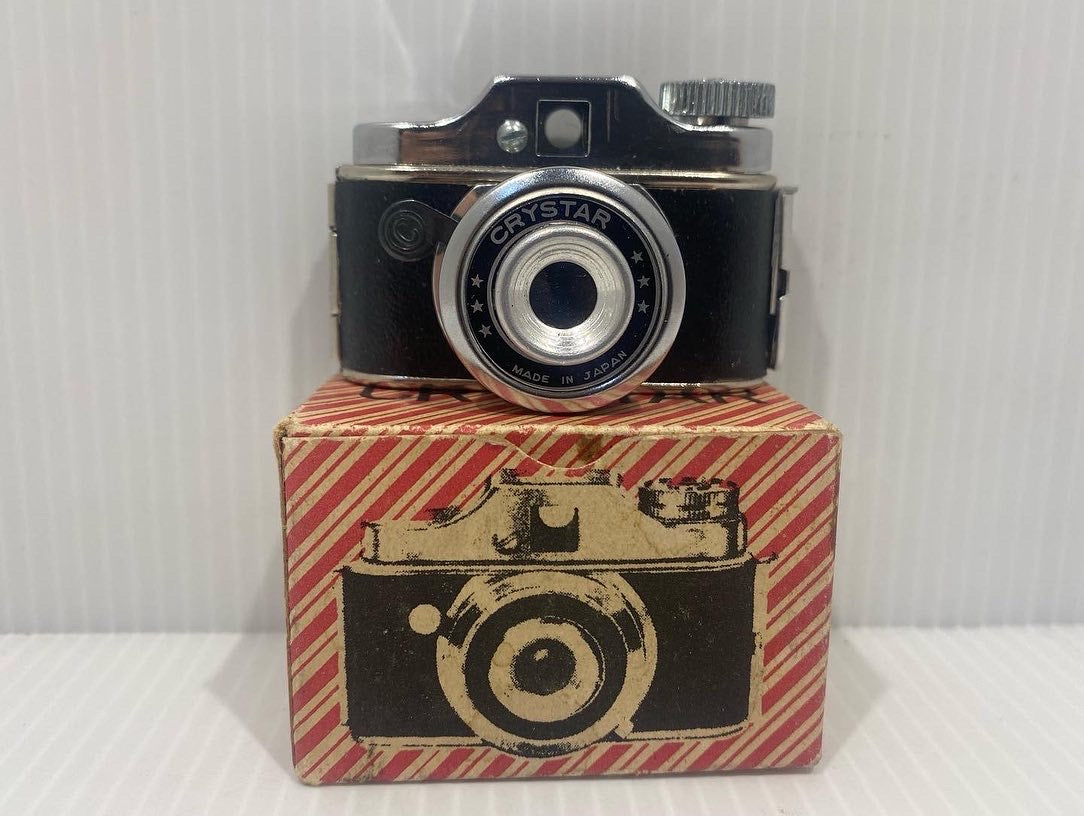The photograph depicts a vintage camera prominently displayed atop its original packaging, set against a background with gray and white solid stripes. The camera is the central focus, featuring a black body and a silver-colored lens. On the lens, the brand name "Crystar" is clearly visible, along with the words "Made in Japan." The camera box below has a striking red and white diagonal striped pattern, reminiscent of a candy cane, and is closed. On the front of the box, there is an illustration or picture of the camera it contained. The camera itself appears to be from the early 60s or 70s, with a large silver knob on the top right, possibly for taking pictures or advancing film, and an additional automatic switch on the front. The detailed and nostalgic presentation suggests that the camera is a treasured piece of photographic history.